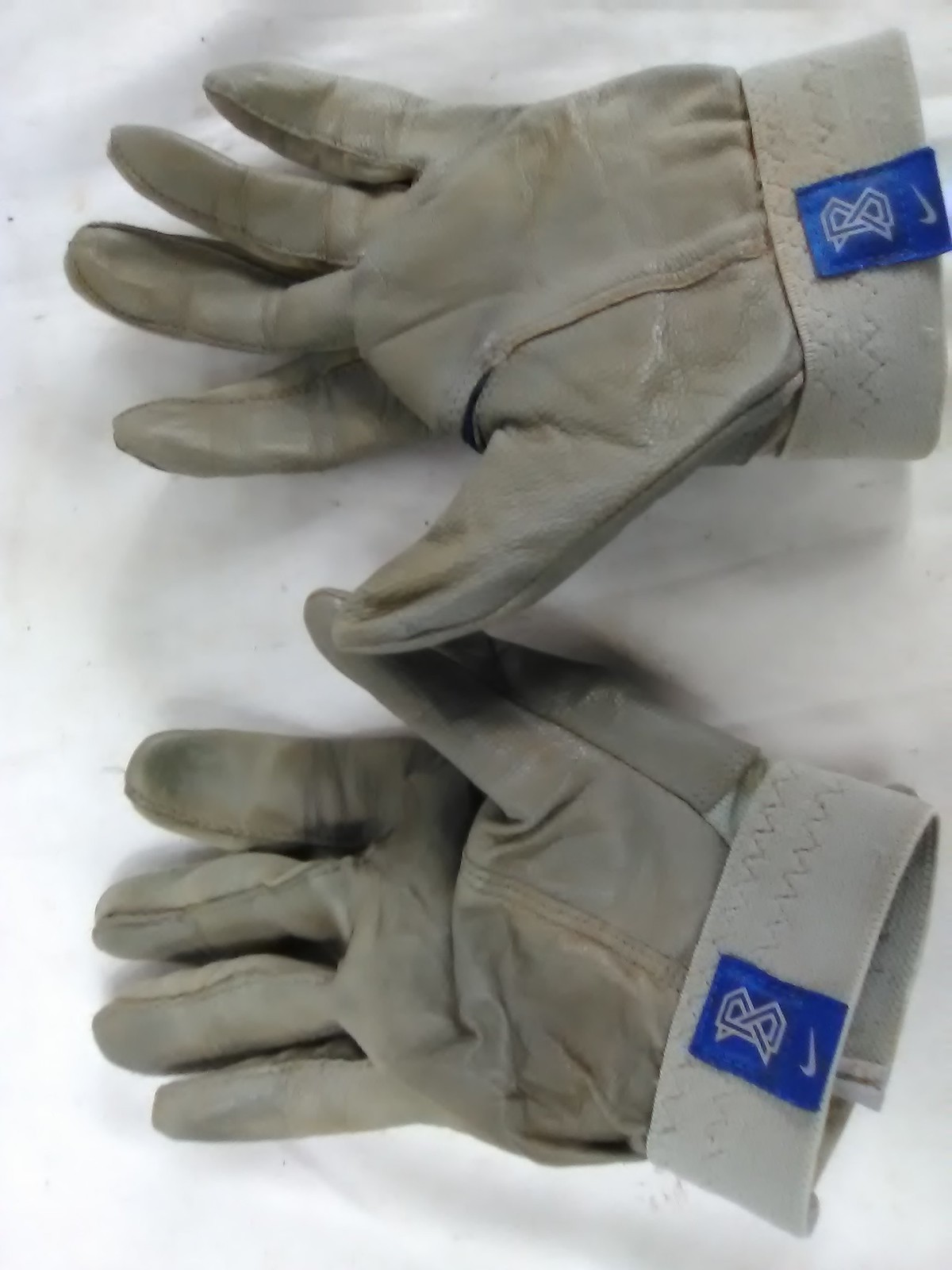This image showcases a pair of worn, sturdy Nike gloves resting palms-up on a white-gray granite-like surface. These gloves, potentially made from leather or suede-like material, exhibit signs of heavy use with visible wrinkles and dirt spots. Their main body color is a dark beige or gray, while the cuffs are a lighter beige or gray and feature a double line of zigzag stitching. Each glove sports a blue rectangular tag on the cuff, displaying the iconic Nike swoosh logo and a B-shaped symbol. The Velcro closure on the cuffs suggests they are adjustable for a secure fit. The right glove appears to need repair, with separation noticed between the thumb and forefinger.